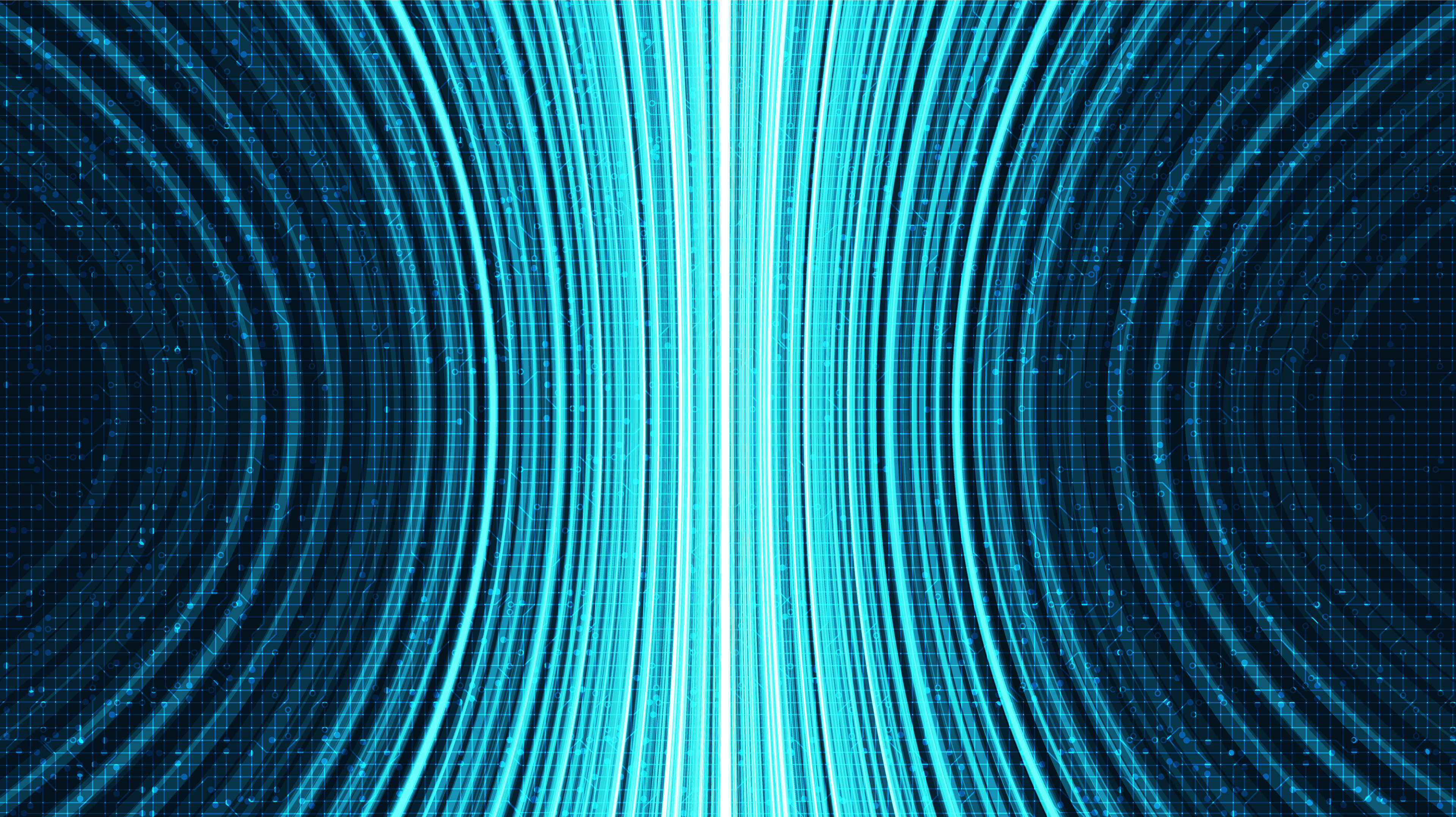The image is a computer-generated graphic featuring a collection of vertical light blue laser lines emanating from the bottom and stretching to the top of the screen. These lines are nearly parallel in the center of the image, which is vividly illuminated in bright blue shades, including darker and lighter blues. As the lines progress outward toward the left and right edges, they gradually darken, transitioning to deep blues and eventually black. Approximately halfway through the image, the vertical lines begin to curve like hyperbolas, forming crescent or semicircular shapes on both sides, with a faint grid pattern overlaying the entire scene. The symmetrical arrangement creates a tunnel-like or mirror effect, and the overall aesthetic resembles digital artwork typical of video games or online media. There is no text present on the image.